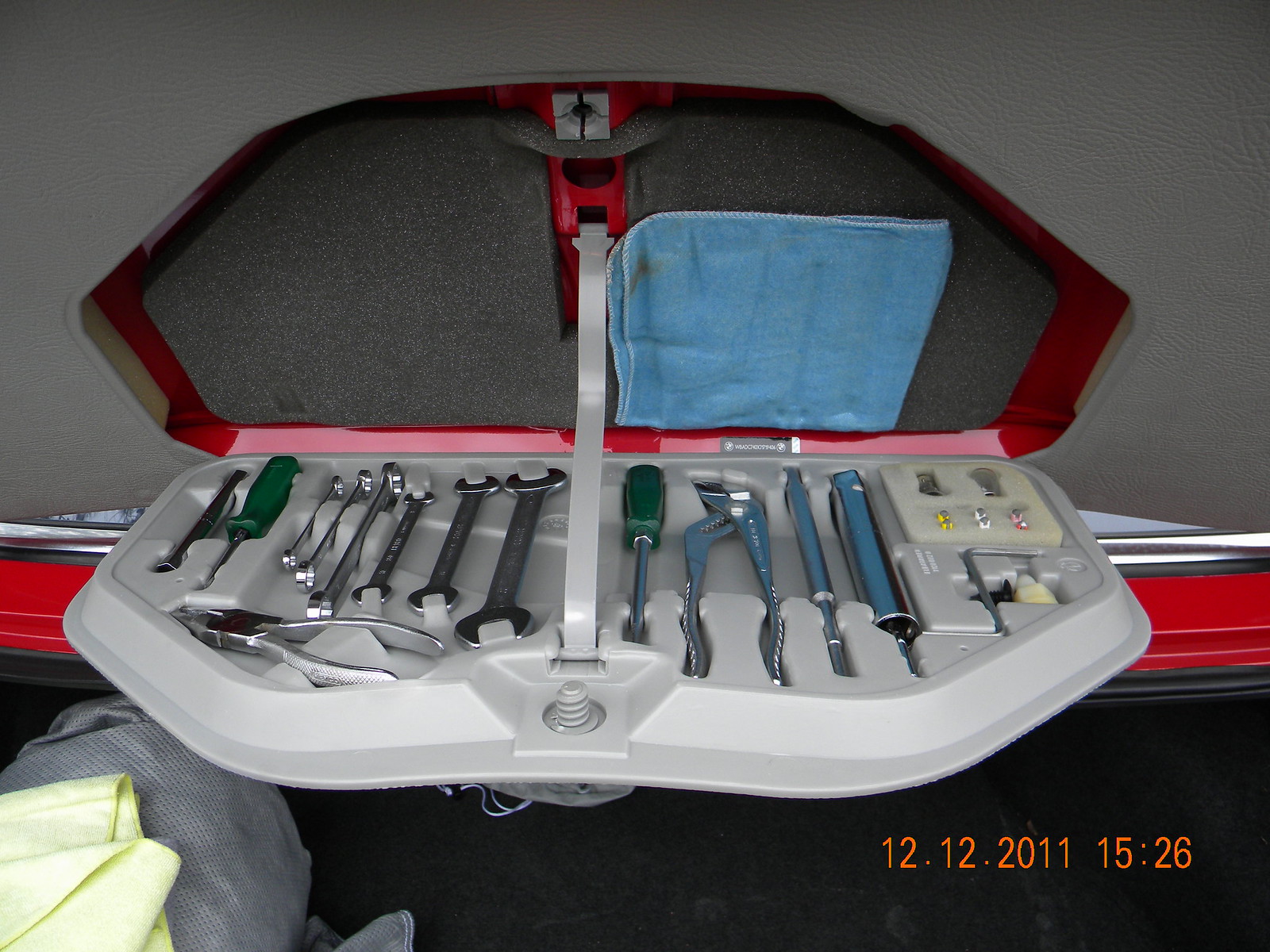The image is a color photograph depicting an open tool case resting on the trunk lid of a red vehicle, with part of the trunk visible in the background. The date "12-12-2011" is displayed in the lower right corner in orange. The tool case has a white bottom and black top, with a blue cloth folded inside the top to protect the tools. The interior of the case features various tools, including a shiny set of chrome wrenches, two green-handled screwdrivers on either side, a socket wrench, crescent wrenches, pliers, vise grips, and possibly some fuses and different colored screws. The tools are organized within individual compartment slots and appear brand new and clean. A gray foam pad cushions the tools inside the case. To the lower left, there is a partial view of a man in a striped shirt, possibly working under the car, though his face is not visible.